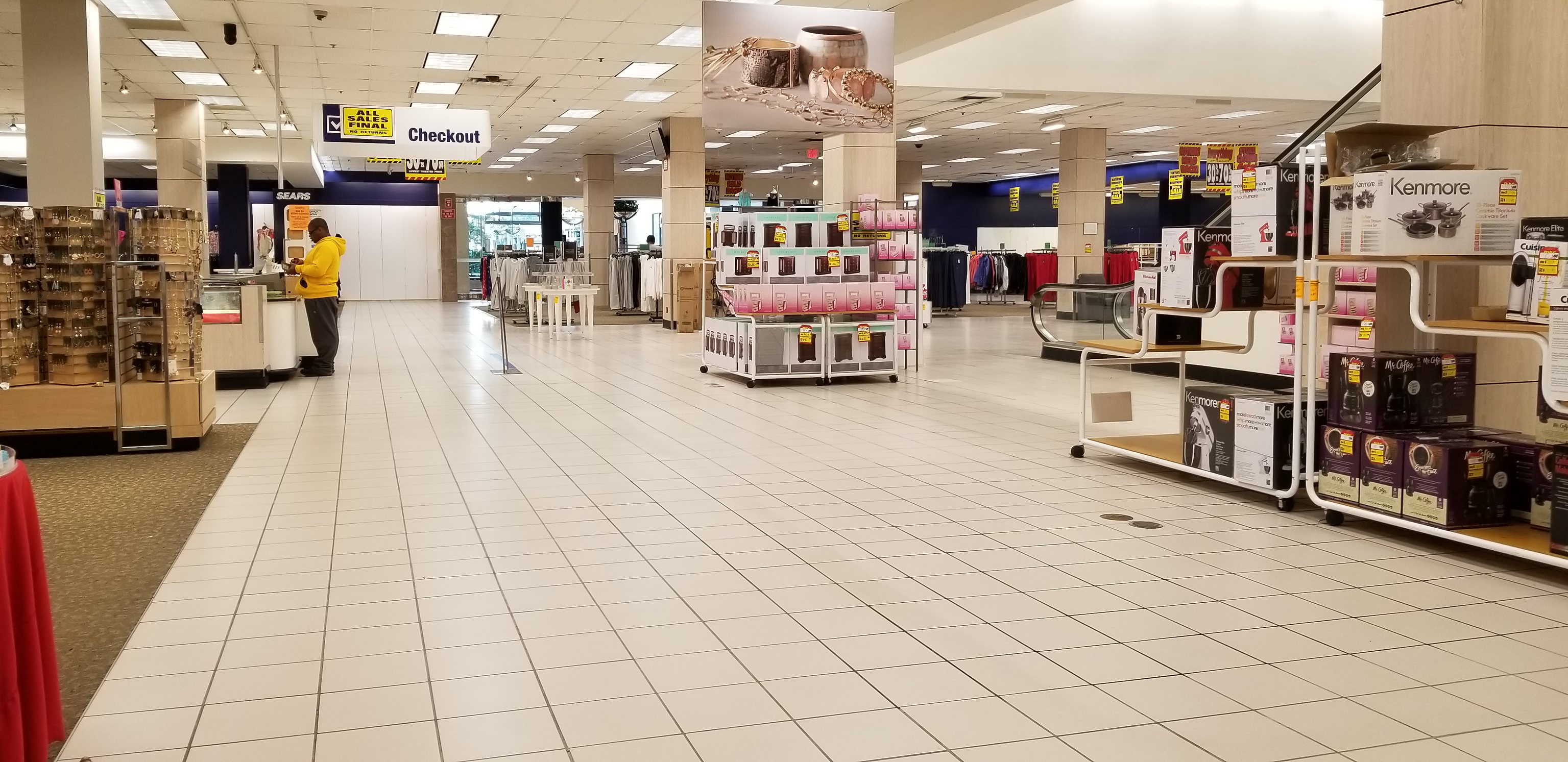A nearly deserted retail store, likely a Sears located in a busy mall, exudes an eerie, uncanny atmosphere with just one visible shopper. The foreground on the left features a white painted, bent metal piping rack stacked with boxes, one prominently displaying a Kenmore cookware set—a Sears trademark. Beyond this display, an escalator with a black handrail and clear glass sides ascends from the mid-background towards the upper right corner. In the far background to the left, racks of clothing are visible. Centered in the image are large square pillars, one adorned with an indiscernible product display. A sign hanging from the suspended ceiling reads "All Sales Final," indicating a checkout area. At this counter stands an overweight man in a bright yellow hoodie and black pants, seemingly in the process of checking out. The white tile floor underscores the desolation, hinting that this Sears store is going out of business.